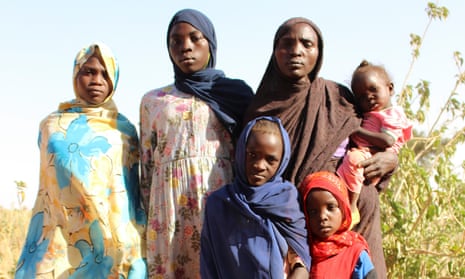The photograph features a vibrant scene of a family standing against a bright blue sky, with some tall green brush visible on the right side. From left to right, the image showcases six black individuals dressed in traditional, colorful garb, perhaps from an African nation. 

The first figure is a young girl wrapped in a blue and yellow shawl adorned with a floral pattern, covering her head and body. Next to her is a woman, possibly her mother, wearing a navy blue headscarf and a pink dress featuring pink, yellow, and green flowers. A young boy stands at the center, swathed entirely in a blue shawl.

Behind him, an older woman, likely the matriarch, wears a red shawl covering her head and most of her body. In her arms, she carries a small child dressed in a pink outfit with yellow shoes. On the far right is another young boy, dressed in a red shawl over a blue t-shirt.

The family exudes a sense of unity and cultural pride, their traditional clothing adding a rich tapestry of colors and patterns to the scene, against the backdrop of the clear sky and wild grass.